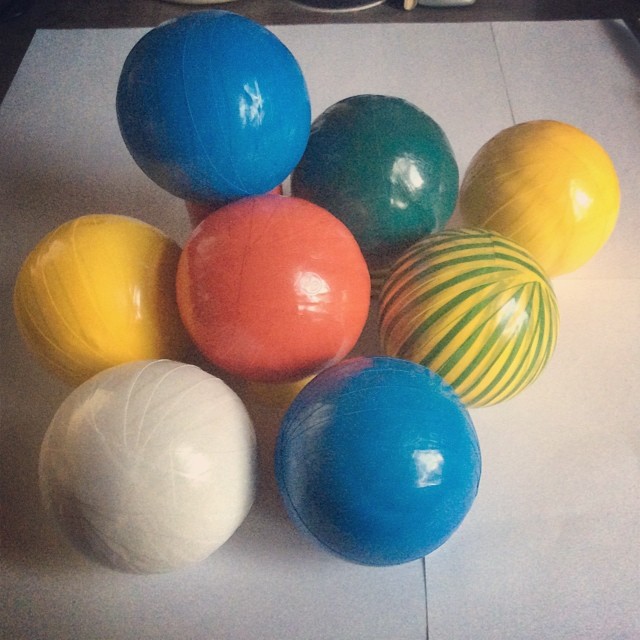The indoor photograph showcases a collection of eight brightly colored, opaque balls, typically used for playground or yard games. Each ball measures about five to six inches in diameter and appears to be made from a material that reflects light, casting shadows to the left due to a light source from the right. They are meticulously arranged on a white, slightly textured surface, possibly paper, with faint black lines visible in the background and a few extending from the top of the frame.

The balls are clustered together but do not form any specific pattern. In the foreground, starting from the lower left, there's a white ball followed by a blue one. At the center, a pinkish or dark peach-colored ball is slightly to the left of a solid yellow ball, with a striped green and yellow ball positioned to its right. The upper left corner features a blue ball elevated on some sort of stand or cylinder, making it appear higher than the rest. Toward the top right, there's a solid green ball, while the yellow ball occupies the extreme upper right corner. The balls display a shiny glare indicative of a camera flash or strong lighting, and they rest on a white backdrop that showcases their vibrant colors. No text or identifying marks are visible in the photograph.